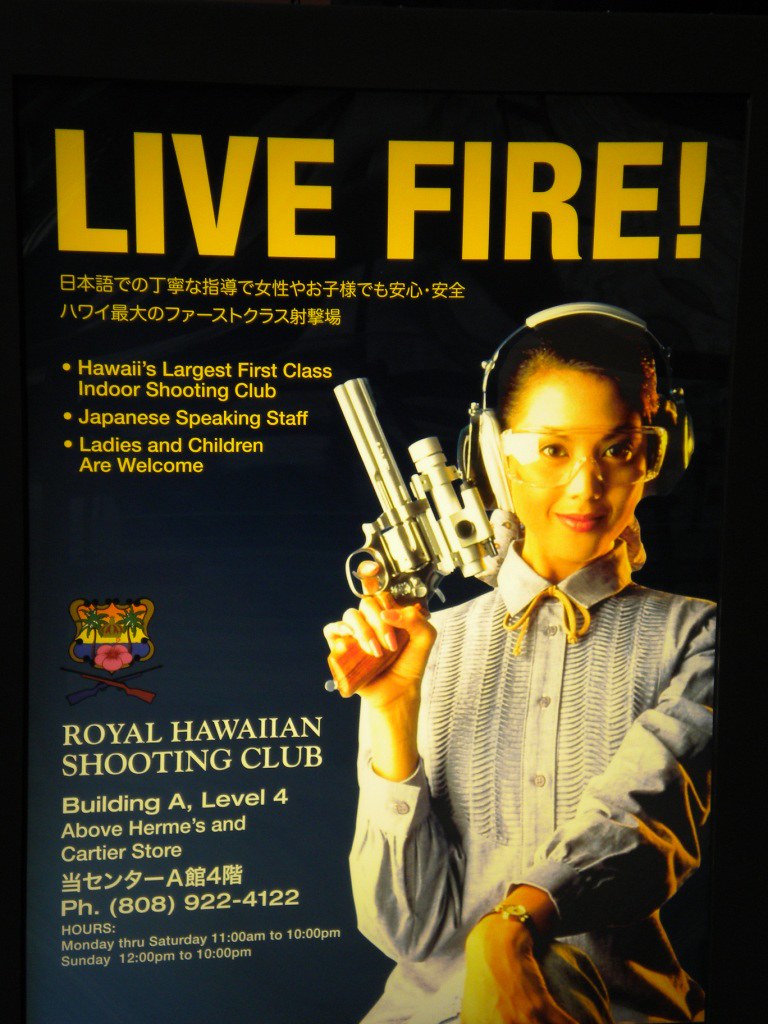The advertisement features a prominent image of a woman dressed in an elaborate, high-necked white dress, complete with protective glasses and earmuffs. Her dark hair is pulled back, and she is holding a large silver revolver with a long barrel and scope attachment, featuring a wooden grip, in her right hand, while her left hand rests on her front leg. The background transitions from black at the top to dark blue at the bottom.

At the top of the ad, large yellow text reads "Live Fire!" Below this, there are two lines of text in Japanese. Following the Japanese text is an enumeration in English that highlights the key offerings of the establishment:
1. Hawaii's largest first-class indoor shooting club
2. Japanese-speaking staff
3. Ladies and children are welcome

To the left of the woman, the advertisement continues with a logo featuring palm trees above a pink flower and a pair of crossed rifles, accompanied by the following details in white text:
- Name: Royal Hawaiian Shooting Club, Building A, Level 4 (above Hermes and Cartier store)
- Address: [Text in Japanese including "A" and "4"]
- Phone Number: 808-922-4122
- Hours: Monday through Saturday, 11 a.m. to 10 p.m.; Sunday, 12 p.m. to 10 p.m.